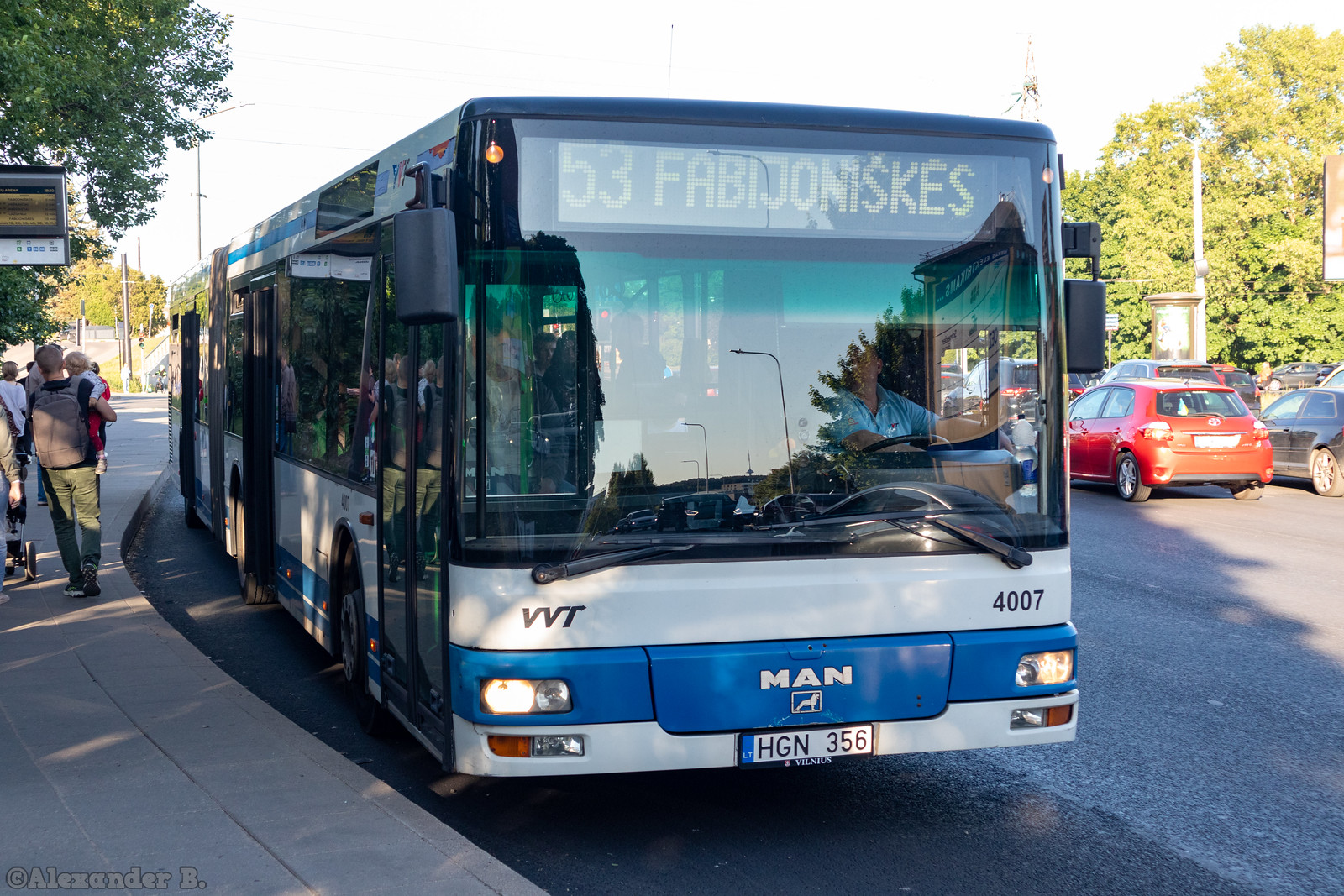The image depicts a white MAN-branded public transportation bus, number 4007, operated by VVT and sporting a blue stripe. The bus, with a license plate reading HGN356, is at a stop in either Finland or Poland, allowing passengers to board and disembark. The digital display on the bus reads "53 FABIJONISKES," indicating its destination. The scene is set on a paved street lined with thick, leafy green trees. Nearby, a red and black car can be seen driving in the opposite direction. The photo captures a pleasant, clear day, with pedestrians, including a man carrying a young child, walking away from the bus.